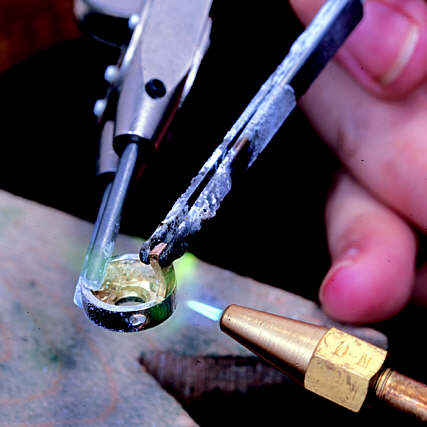The image depicts a close-up scene of someone engaging in precise soldering work on a small metal object, potentially a ring, using a delicate welding tool. The welding tip, golden in color, emits a small, intense blue flame. The individual's hand, appearing pinkish-tan and positioned near the flame, skillfully maneuvers industrial tweezers holding the metal piece, which seems to be melting under the heat. A secondary silver tool is also in use, contributing to a green glow, likely caused by a chemical reaction. The background is blurred and black, contrasting sharply with the focused, intricate work being performed. The work surface underneath the metal object is light-colored and mottled, adding further detail to the close-up nature of the image.